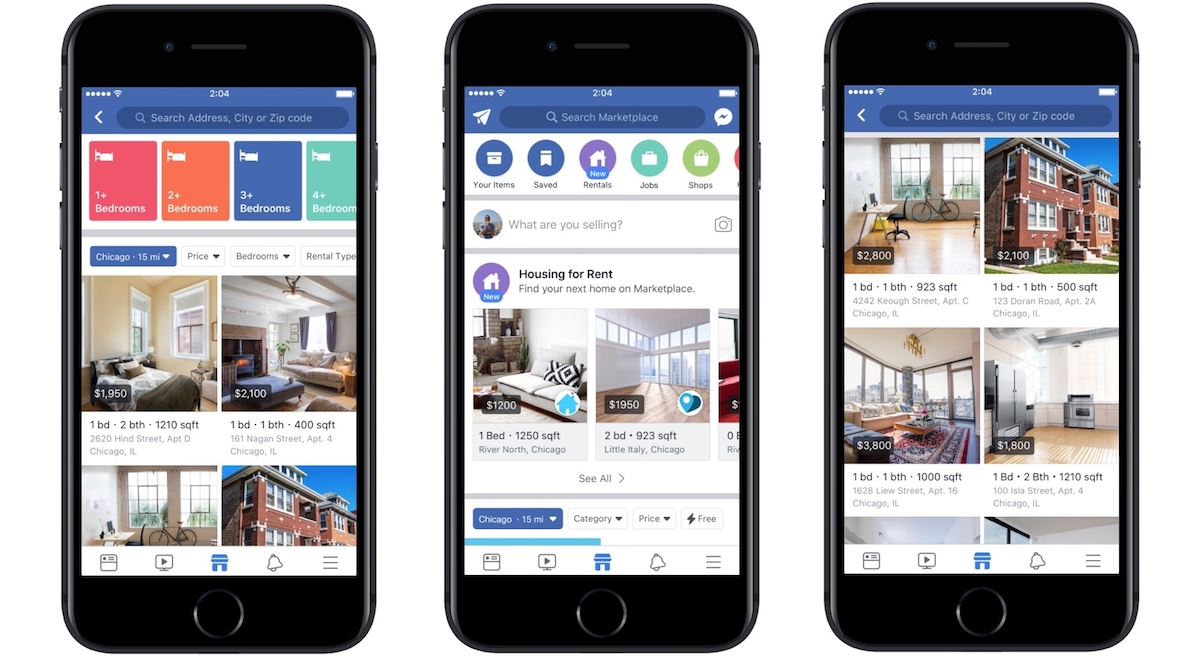The image displays three smartphones positioned side by side. Each phone screen shows a similar interface, featuring a blue banner at the top with five white dots, a Wi-Fi icon, the time reading "2:04 PM," and a fully charged battery icon. The middle phone has an additional send arrow icon and a messenger signal icon flanking its search bar.

The first phone screen is focused on a housing rental app. It features a segmented area showcasing four colored sections, each representing different bedroom counts from one to four. Below this, there is text that partially reads "Chicago 15" and an arrow suggesting a dropdown option. Four image thumbnails of residential interiors are displayed, two of which are partially visible. These images detail bedrooms with accompanying size information.

The middle phone screen also displays a housing rental app. Underneath its search bar, there are icons including a person icon and a profile symbol suggesting user interaction options like "What you're selling." The screen shows listings for housing rentals, including information on pricing, the number of bedrooms, and partially visible additional details. The bottom of this phone screen displays "Chicago 15 miles" alongside a blue button on the right-hand side. There are six images in total, though only four are fully visible, each featuring residences with details like pricing, bedroom and bathroom count, square footage, and supplementary information.

Each phone screen in the image is designed to facilitate a comprehensive user experience for searching housing rentals, providing detailed visual and textual information for potential renters.